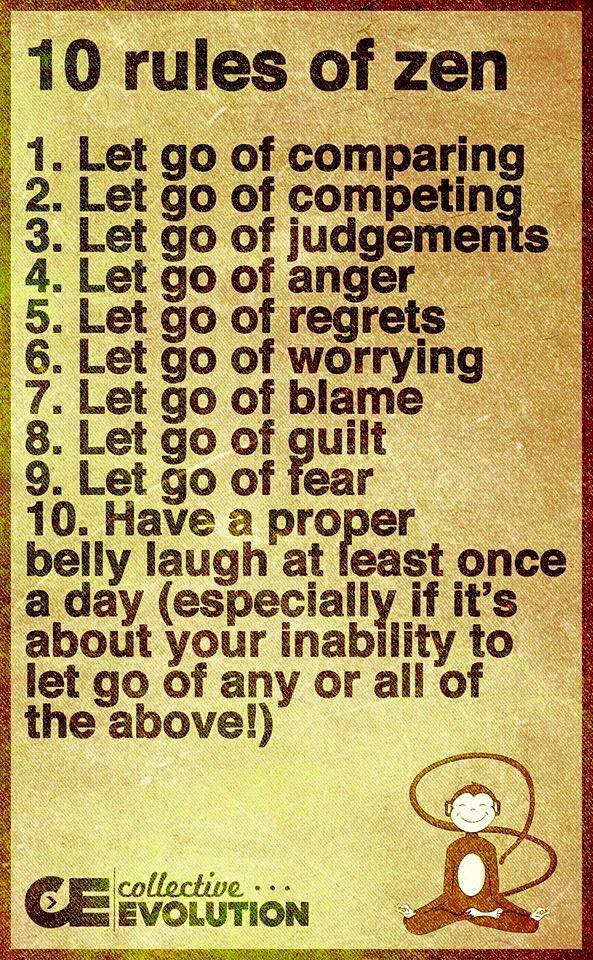This printed image features a tan background with a brown frame and is designed vertically. At the bottom right corner, there is a cheerful brown monkey with a long tail and a smiling expression. Next to the monkey, the logo "CE" representing "Collective Evolution" is displayed. The primary text in black letters at the center of the image lists "The 10 Rules of Zen," which include: 1. Let go of complaining, 2. Let go of competing, 3. Let go of judgments, 4. Let go of anger, 5. Let go of regrets, 6. Let go of worrying, 7. Let go of blame, 8. Let go of guilt, 9. Let go of fear, and 10. Have a proper belly laugh at least once a day, especially if it’s about your inability to let go of any or all of the above. The serene and contemplative setting, complemented by the meditating monkey, visually emphasizes the essence of mindfulness and letting go.